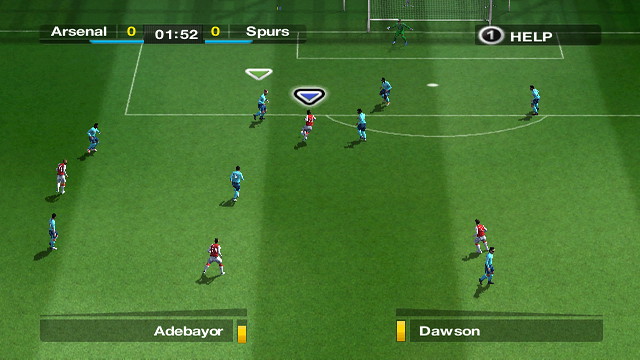In this image, a scene from a soccer video game is depicted. The virtual match features players from two teams identifiable by their jerseys: most players are wearing blue jerseys, while a few are dressed in red. The action is concentrated near the goal area, where a goalkeeper, wearing green, stands in front of a net framed in white.

Several white lines marking the field can be seen under the players' feet, providing a clear sense of the soccer pitch layout. Near the center top of the image, a couple of players have icons above their heads: one has a grayish upside-down triangle, while the other player has a similar icon marked in blue with a black border.

The user interface (UI) of the game is visible at the top of the screen. On the left side, it displays "Arsenal 0 - 0 Spurs" along with the match time of "52:01". The top right corner of the screen shows a "Help" button. At the bottom left, the name "Ade Bayor" is displayed, while the bottom right shows "Dawson", both names accompanied by small yellow bars beside them.